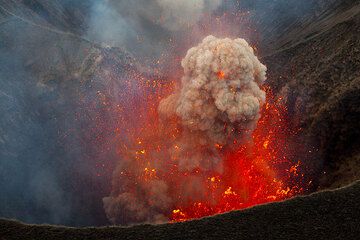This photo captures a dramatic volcanic eruption viewed from the rim of the caldera. In the center, vibrant, molten lava in shades of dark red, orange, and yellow spews explosively upwards, tracing a path from the bottom right towards the top. A gigantic plume of smoke and ash dominates the scene, emerging from the heart of the eruption and blending into the varied gray hues of the sky. The foreground reveals the dark, rugged edges of the volcanic rim, seen from above as if the viewer is peering directly down into the caldera. The surrounding landscape consists of dirt and rock, their muted tones highlighting the fiery center. No text distracts from the raw power of nature displayed in this zoomed-in shot, encapsulating the intense, dynamic energy of a volcanic explosion.